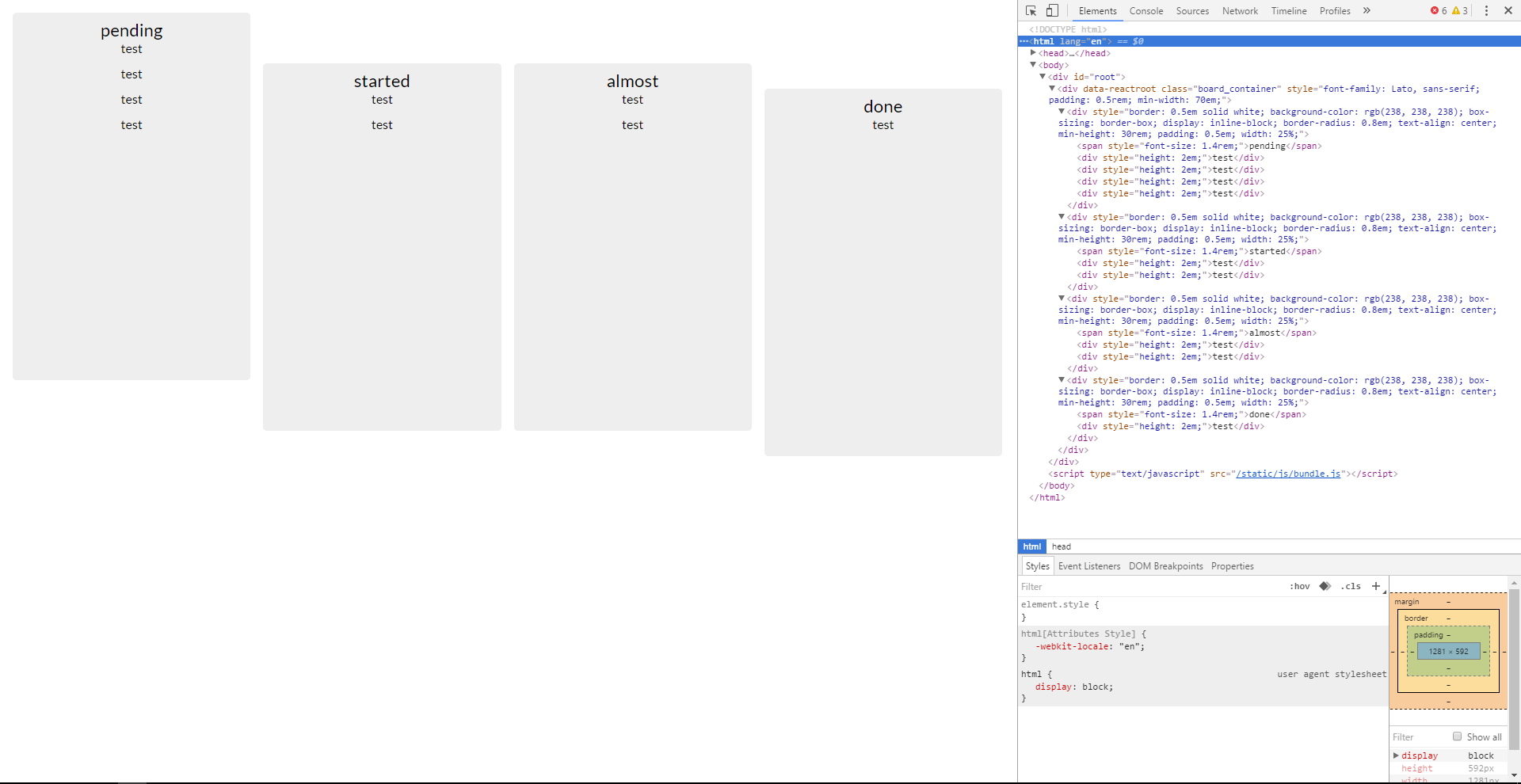The image displays a computer screen with a specific focus on a section featuring four distinct boxes positioned vertically on the left side. The first box, slightly elevated, has a gray background with the word "Pending" prominently centered in black text. Beneath the word "Pending," the word "test" is listed four times in consecutive rows.

Next to the "Pending" box are two equally sized boxes aligned horizontally. The first of these boxes is labeled "Started," with the word "test" appearing twice underneath in descending order. Adjacent to the "Started" box is another one labeled "Almost," similarly containing the word "test" twice beneath it. 

The final box is positioned slightly lower than the "Started" and "Almost" boxes, creating a visual offset. This box is labeled "Done," with "test" written once directly below the label.

Additionally, the screen features a developer tools interface at the top, which includes various tabs labeled "Elements," "Console," "Sources," "Network," "Timeline," and "Profiles." Below these tabs, a section displays a collapsed arrow indicator along with "!DOCTYPE html" and an arrow. A blue headline reads `<html lang="en">` and is followed by text including `== $0`. Beneath this are multiple lines of printed code or text details.